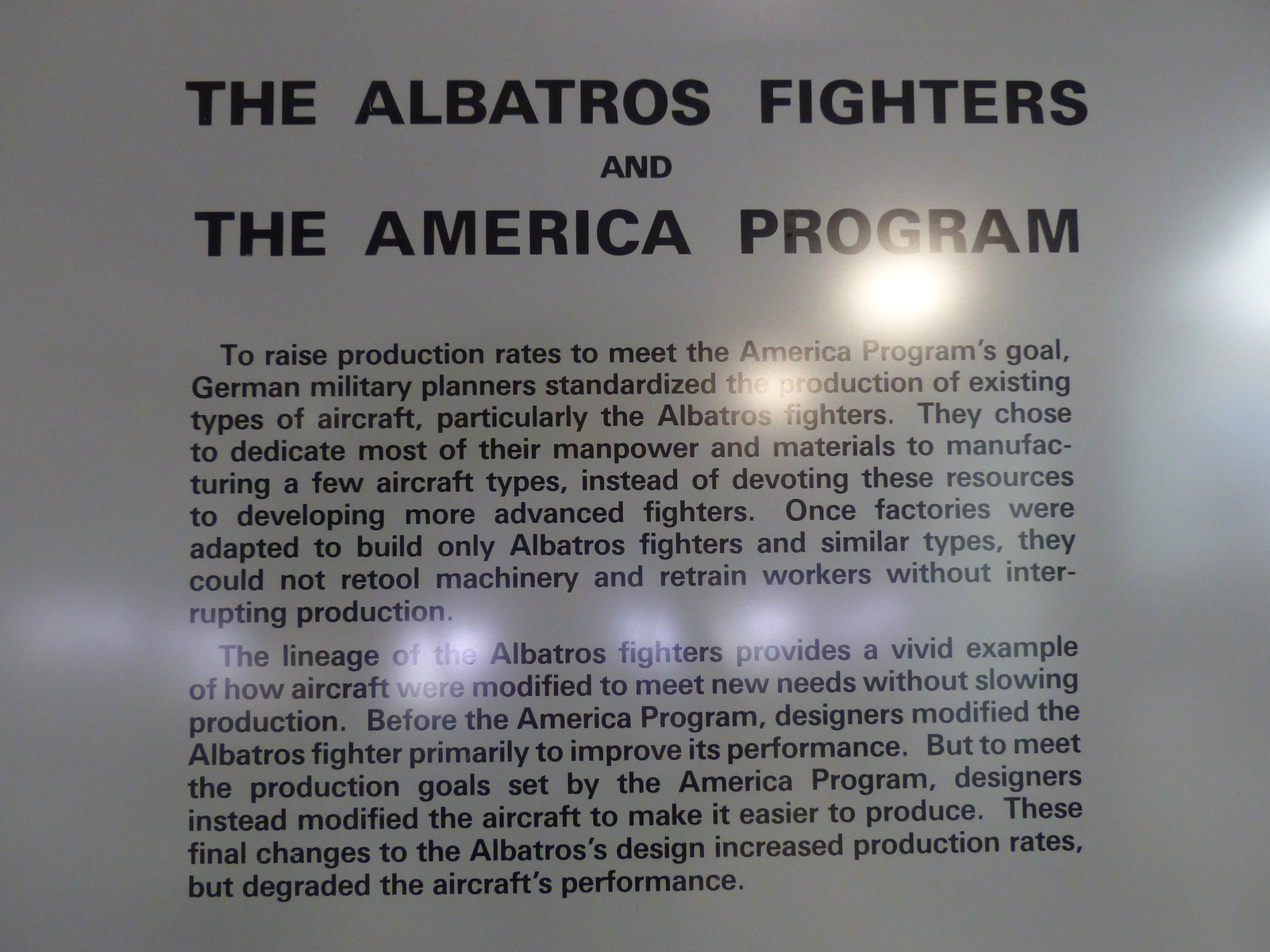This image showcases a reflective, possibly metallic or acrylic, museum display label encased in glass. The background is a grayish-white with black text, presumably in a Helvetica font, and is situated in an indoor setting with visible glare from windows and light bulbs. The display is titled "The Albatross Fighters and the America Program." It contains two paragraphs detailing how German military planners standardized aircraft production to meet the America Program’s goals by focusing resources on manufacturing existing types, particularly the Albatross Fighters. Despite the streamlined production increasing output, it hindered the development of more advanced fighter planes and degraded the aircraft's performance due to the simplified modifications aimed at easing production processes.